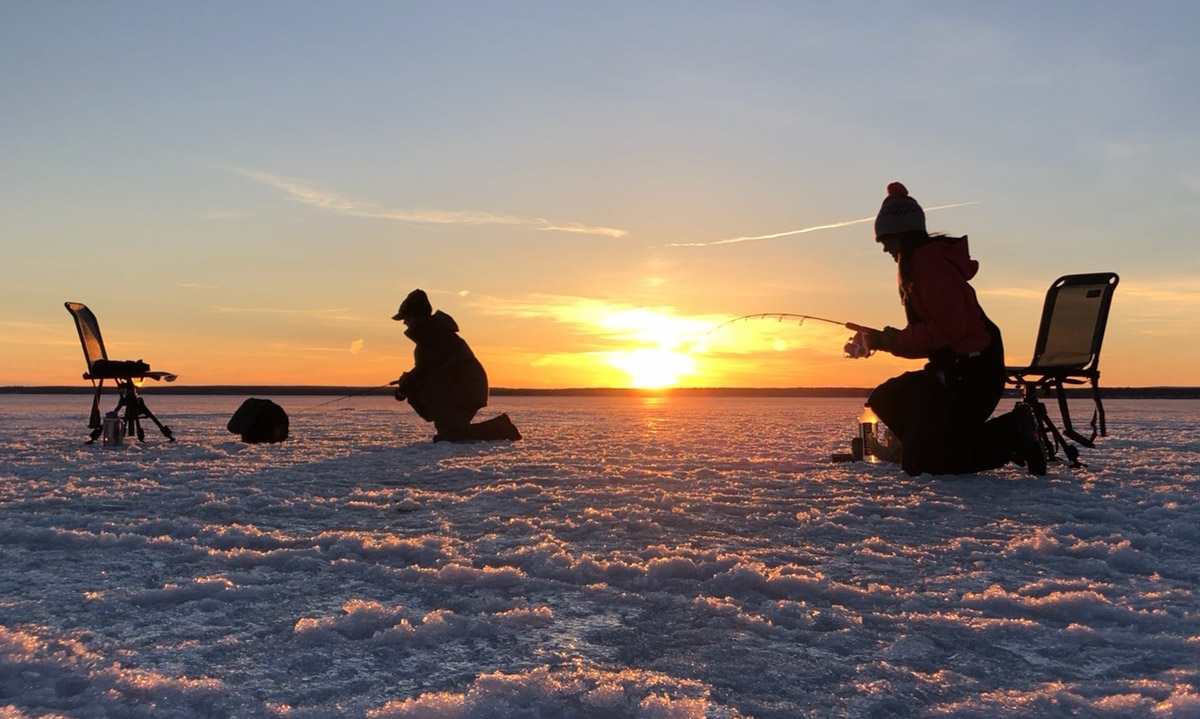In this outdoor image, there are two people ice fishing on a snow-covered beach. They are kneeling on the ice with their fishing poles extended into the water. The beach, although typically not associated with snow, is entirely covered in it, suggesting a cold winter setting. In the background, the sky displays a beautiful, though distant, sunset, casting light over the barren landscape and adding a serene glow to the scene. The ice fishermen are dressed warmly in pants and jackets, with one wearing a ski hat and the other a baseball cap, indicating the chilly conditions. There are two chairs placed nearby on the icy surface, and a few clouds are visible in the sky, contributing to the overall quiet and cold atmosphere of the picture.